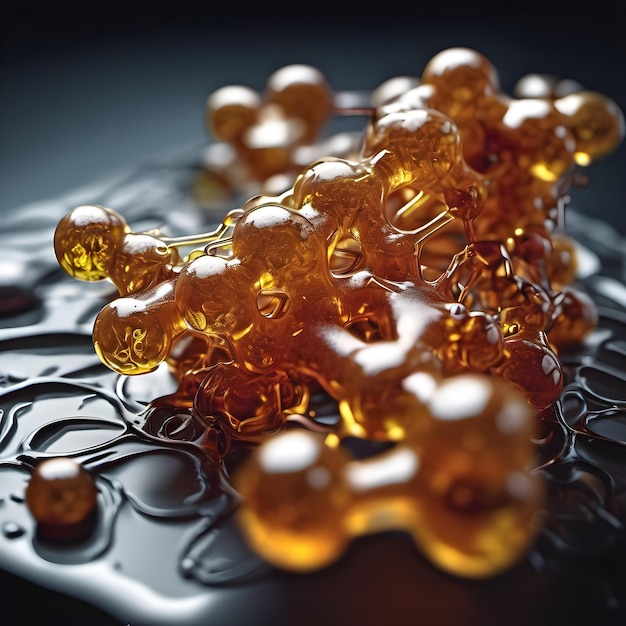This close-up, abstract photograph, rich in gold and amber tones, features an arrangement of spherical, honey-colored globules of varying sizes. These globules, appearing as though they are thick droplets of liquid, either connect with thin cylindrical strands or rest independently on a highly textured, dark gray surface. The light source is artificial, illuminating parts of the globules and surface, creating a glossy, reflective sheen. The black surface beneath them shows oily, stained patterns from the liquid, adding to the overall texture. In the image's corners, especially the upper left and right, there is an absence of light, creating a stark contrast with the illuminated middle section. The globules appear interconnected in some areas, resembling tiny dumbbells coated in an oil-like substance. The surface they rest on is visible in certain segments, curving and disappearing behind the globules, with lighter edges highlighting their contours.